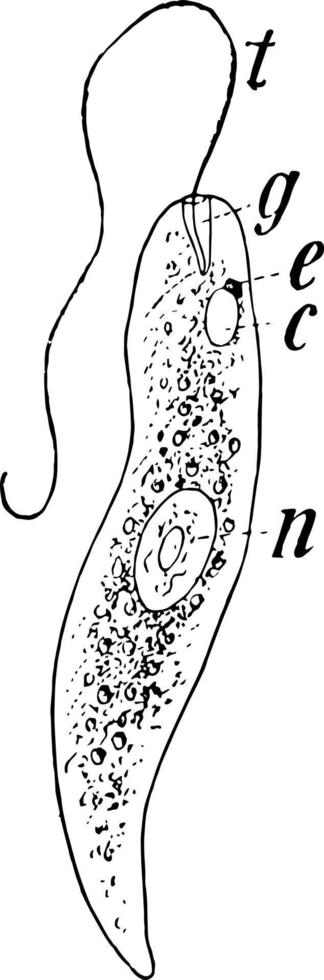The black and white illustration depicts an organism-like shape resembling a paramecium or a chili pepper, with a bulbous top tapering into a pointed bottom. The figure features a wavy, snake-like antenna labeled with the letter 'T' extending from the top left side. The main body of the blob is characterized by numerous small circles and dots. The central part contains a distinct circle labeled 'N' for Nancy. Surrounding this central circle are various other labeled sections: 'G' marks the top of the blob, 'E' is situated slightly below 'G,' and 'C' is further down. The neat, white background contrasts sharply with the black, line-drawn elements, giving the illustration a crisp, clean appearance despite its complex, somewhat chaotic detailing.